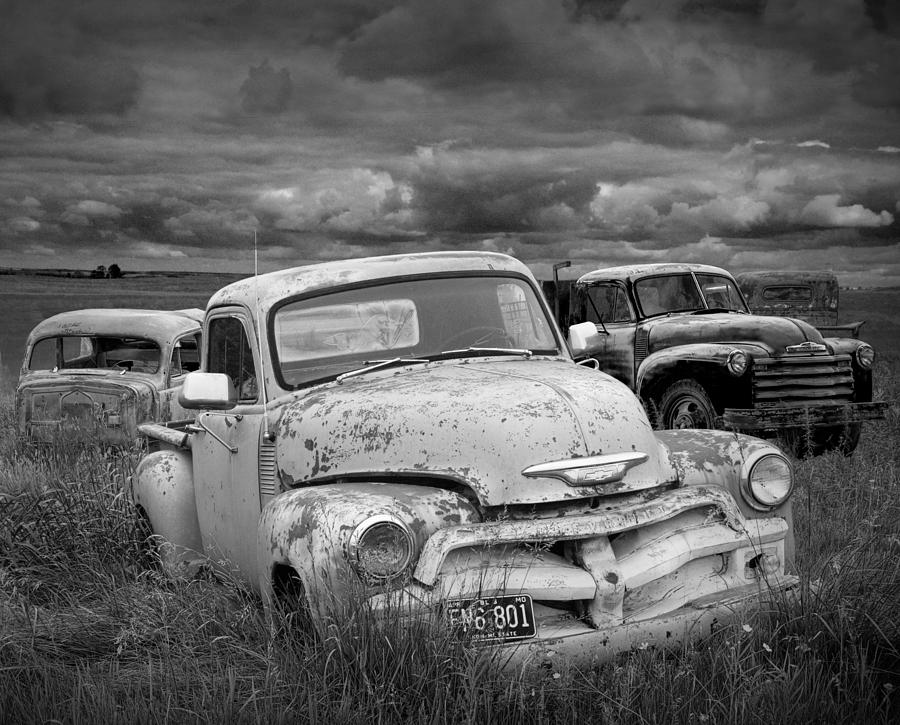This professional black-and-white landscape photograph captures a poignant scene of abandonment and decay. The main focus is a group of four vintage, rusted cars, presumed to be Fords, scattered haphazardly in an overgrown field. The cars, which have largely lost their paint to rust, are enveloped in tall grass that obscures their tires and reaches up to their headlamps. The front car, centrally positioned, has its hood popped open, revealing the license plate with the number FN6801, from Maryland. These empty, antique vehicles, which include a possible truck, present a stark contrast against the well-mowed field in the background.

Above this tableau, the sky occupies the top third of the image, filled with swirling, tumultuous clouds in varying shades of gray and black. The ominous, dense clouds hint at an approaching storm, though a sliver of sunlight tries to pierce through the gloom. The absence of buildings or other structures emphasizes the isolation and desolation of the scene, making it a powerful, evocative snapshot of forgotten relics quietly deteriorating in a neglected field.